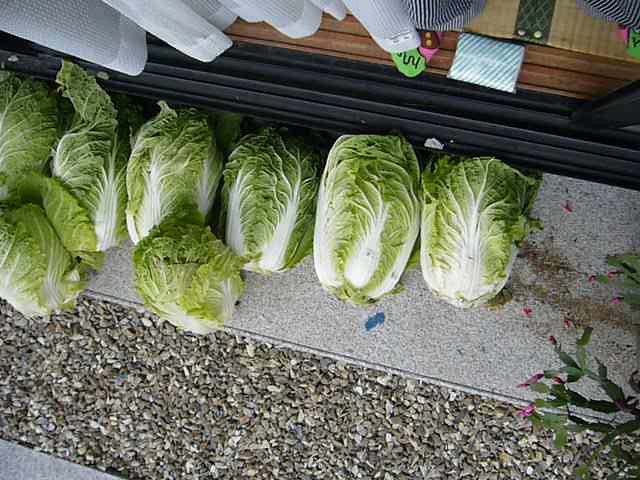This is a detailed aerial photograph of eight Napa cabbages lined up side-by-side on a light grey concrete pavement outside a doorway. The cabbages are vibrant green with distinctive white veining and firm white cores. Below the pavement, there's an area scattered with rocks in shades of light brown, brown, and grey. On the bottom right corner of the image, a plant with green leaves and small purple flowers peeks into view. Behind the cabbages, you can see a black and brown doorway threshold, partially covered by white curtains with vertical lines. Additionally, there is a blue object on the pavement in front of the second cabbage from the right, and in the top left, a white object with diagonal grey lines and a green object with black lines are visible.